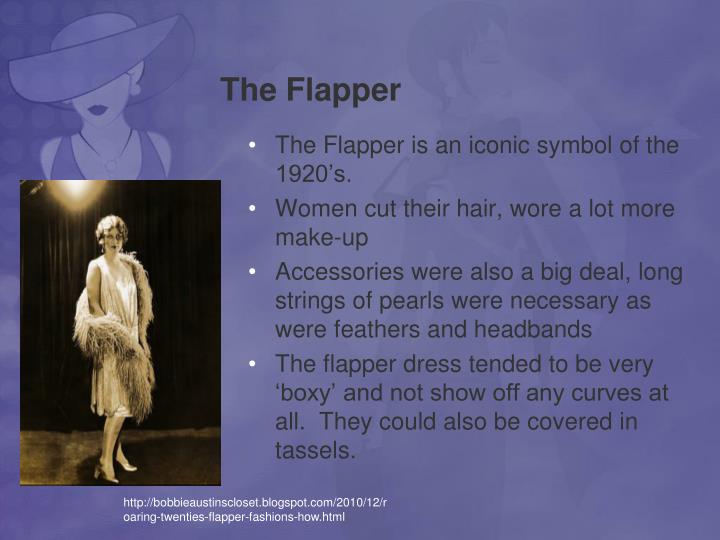The image features a predominantly purple background adorned with various figures. The central focus on the left is a woman integrated into this purple setting, distinct by her fancy hat, earrings, lipstick, necklace, and a shirt. The shirt transitions into an authentic historical photograph from the 1920s, presenting a young woman in black-and-white attire, complete with a fur-like scarf draped around her, silver or white shoes, and a white dress. She stands on a solid floor with a plush carpet behind her, stage lights and a dark curtain in the background accentuating her performance setup. 

On the right, a faint, cartoon-like male figure also in purple attire, facing right, adds depth to the image. The visual is an educational slide titled "The Flapper," highlighting this iconic 1920s symbol. Bullet points detail the hallmark features: short haircuts and increased makeup usage by women, essential accessories like long strings of pearls, feathers, and headbands, and the flapper dress itself, which was notably boxy and often adorned with tassels to hide any curves. The visual elements suggest the image emanates a sepia tone and there is a link in white at the slide's bottom, adding a final modern touch.